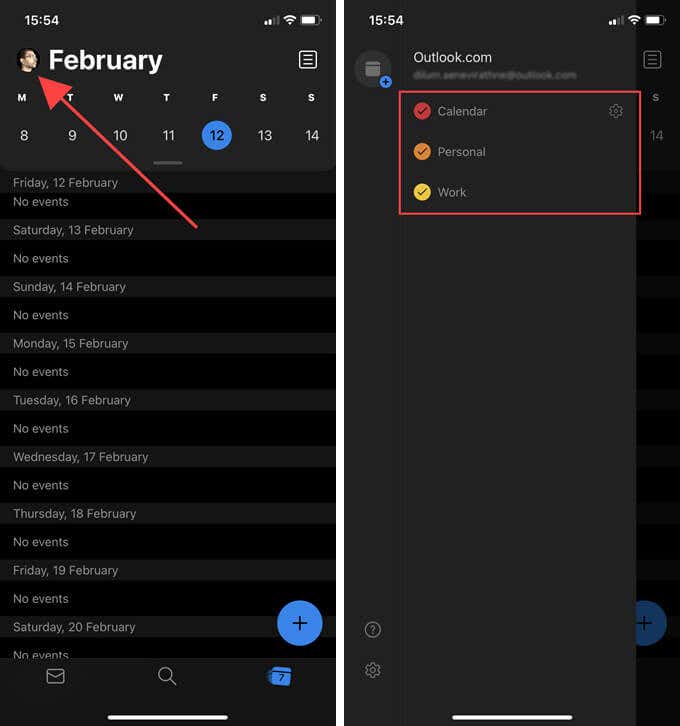The image consists of two side-by-side screenshots taken from a smartphone, likely an Android device. Both screenshots are in dark mode, adorned with dark gray and black backgrounds depending on the specific section.

The first screenshot on the left exhibits a typical status bar at the top, showing the time as 15:54, signal strength icons, Wi-Fi signal strength, and a partially depleted battery icon. Beneath this status bar is a calendar interface displaying a list of events. Prominently, a small round avatar, presumably the user's photo, is situated next to the word "February." Adjacent to this is a list icon symbolizing a text document with lines.

Days of the week (M, T, W, T, F, S, S) are visible across the calendar, with the dates 8 to 14 beneath them. The date "12" is particularly highlighted in blue, making it stand out. Further down the calendar, specifically on Friday, the 12th of February, it is noted that there are "no events," a pattern repeated through Saturday, the 20th. At the bottom center of the screen, there's a round blue button featuring a plus sign, likely designed for adding new events. The bottom navigation bar includes icons resembling an envelope, a magnifying glass, and a calendar with a question mark.

The second screenshot, just to the right, shows an interface from Outlook.com. A red rectangular box highlights three options: "Calendar," "Personal," and "Work." Each option is accompanied by a distinct colored button: red for Calendar, orange for Personal, and yellow for Work, all marked with check marks. A prominent red arrow, likely an annotation, points towards the user's photo in the first screenshot, suggesting it might not be a part of the original interface but added for illustrative purposes.